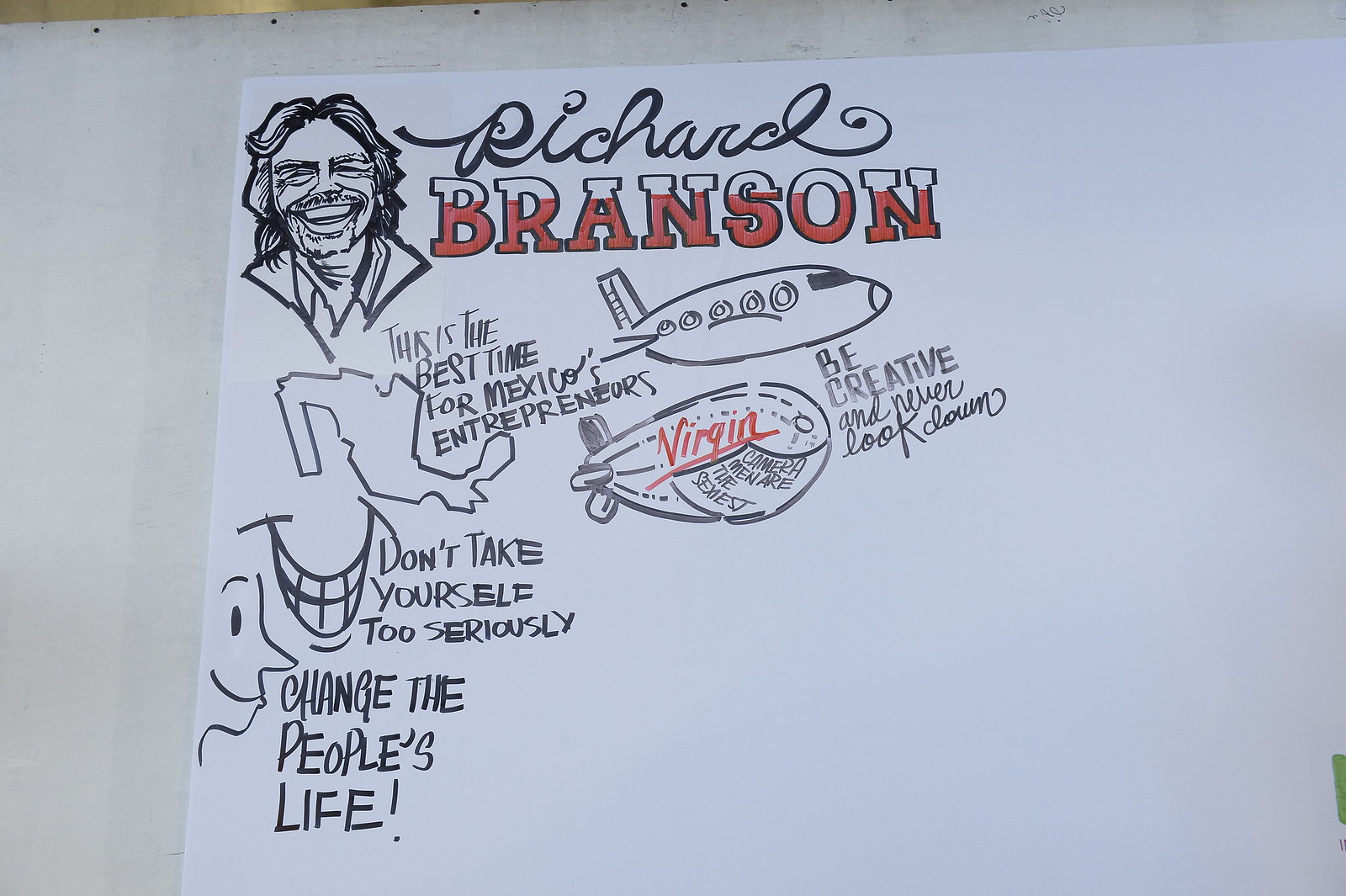The image features a sheet of paper with various drawings and text, positioned against an off-white background. Dominating the upper left corner is a caricature of Richard Branson, easily identifiable by his big smile, bushy eyebrows, long hair, and a collared shirt. To the right of his caricature, his name is written; "Richard" in cursive black, and "Branson" in large blocky letters with the bottom two-thirds colored red.

Beneath the caricature, a series of motivational quotes and drawings are spread across the page. The text "This is the best time for Mexico's entrepreneurs" appears next to an outline of the country of Mexico. Adjacent to Mexico, there is an illustration of a blimp with "Virgin" written in red on its side and a drawing of an airplane above it. Below this, the text states, "Be creative and never look down."

Further down, a cartoon-like smiley face is accompanied by the phrase "Don't take yourself too seriously." Nearby, there is a profile sketch of a person, simply drawn with a smile, long nose, and a single eyebrow, beside the encouraging words "Change the people's life."

The entire composition appears to be a personal sketch or poster, likely created indoors, possibly in someone's home. The predominant colors in the drawing are black, red, gray, and shades of white and off-white.